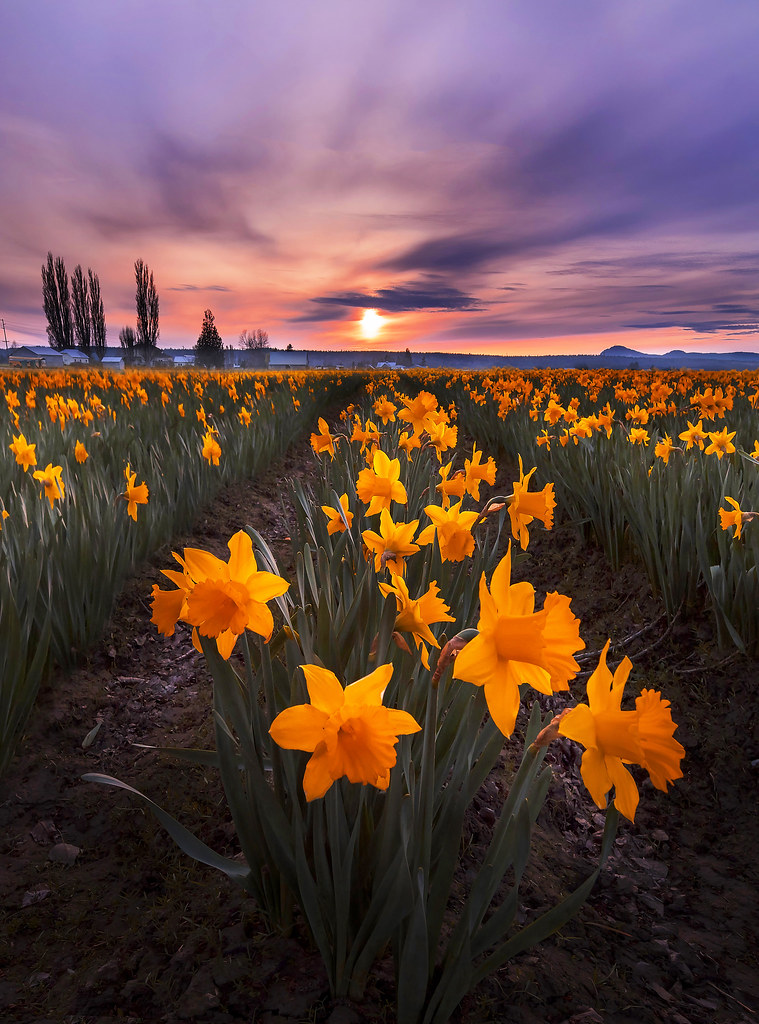This vibrant, computer-generated image captures an expansive field of bright yellow marigold flowers, meticulously planted in neat, parallel rows that stretch far into the distance like an endless sea of gold. Each marigold is perched atop a long, slender green stalk, creating a harmonious contrast against the horizon. The scene is framed by a stunning sunset, where the sky transitions from dark purple at the top, through a gradient of pink and orange hues, to a faint blue near the horizon. Low-lying, dark clouds hover above, while the dimming sun casts a serene glow across the landscape. Far in the background, quaint white farming houses and distant mountains can be seen, adding a touch of rustic charm. Tall trees on the left and a hint of high ground on the right complete this picturesque panorama.